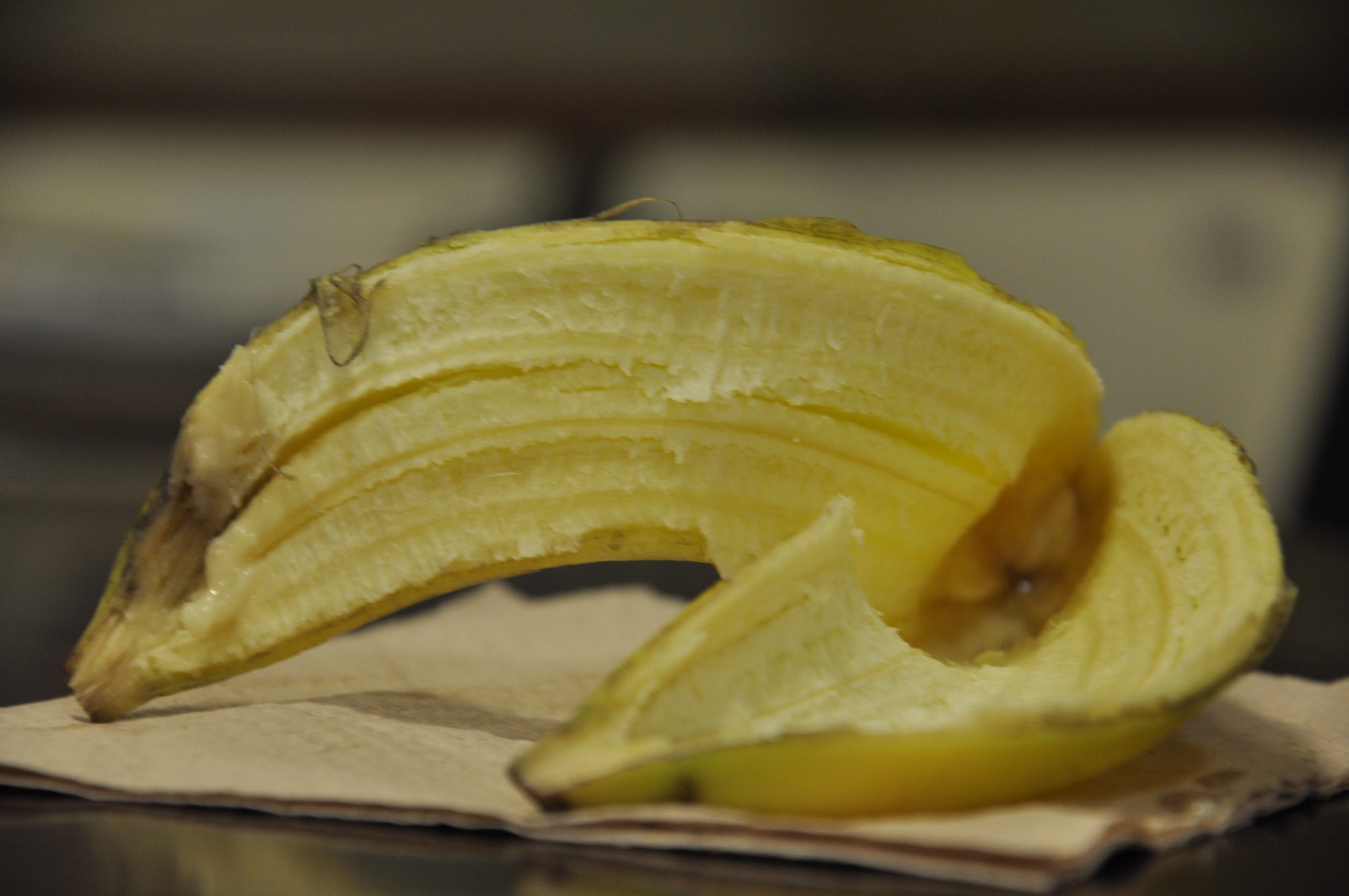The image showcases a yellow banana peel, prominently positioned atop a neatly folded white paper towel, which itself rests upon a table. The vibrant banana peel, which retains only a small amount of banana flesh near its middle, starkly contrasts with the paper towel. The paper towel appears to be folded at least two or three times, providing a layered cushion for the peel. The background of the image is intentionally blurred, with faint glimpses of two red chairs and indistinguishable elements, drawing focus entirely on the subject. A subtle shadow cast by the peel adds depth to the composition, highlighting the textures of both the peel and paper towel.